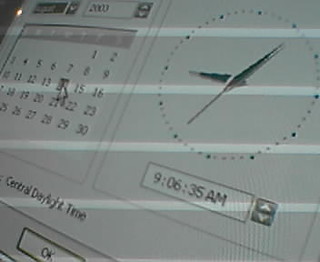The indoor photograph depicts an angled view of a computer display featuring an older date and time settings program. Dominating the upper right of the screen is an analog clock face without numbers, only dots, showing the time at 9:06 AM. Directly beneath the clock, a digital readout precisely marks the time as 9:06:35 AM, accompanied by arrow buttons for adjustments on the right.

On the left side of the screen, the calendar settings are visible, with the cursor highlighting the date '14' in the foreground. The background of the display is white, with all text and elements rendered in black. 

Additional details include the text "Central Daylight Time" diagonally positioned in the bottom left and part of a rectangular "OK" button peeking out from the lower right corner. Aesthetic elements of the photograph include four evenly spaced, light white vertical lines that traverse the entire image. The overall appearance and design suggest the software belongs to an older era of computer applications.